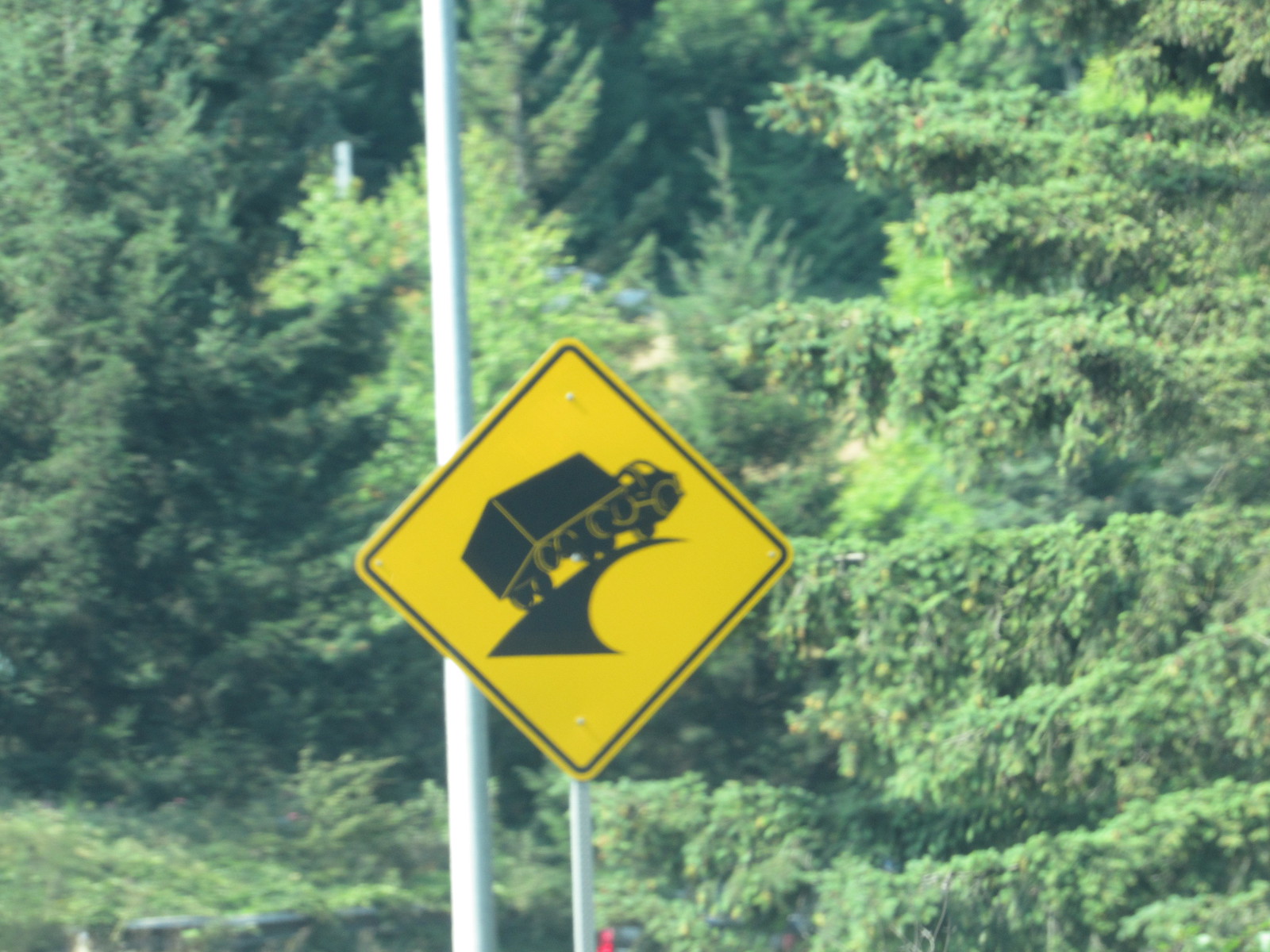This detailed horizontal image captures a yellow diamond-shaped warning sign with a black border, prominently displayed on a silver pole. The sign features a small semi-tractor trailer truck at an angle, signaling a tipping hazard on an upcoming sharp curve. The background reveals lush greenery, including pine trees, shrubs, and vining plants, against a hillside. A tall white lamp post stands to the left of the center, extending from the bottom to the top of the frame, partially cropped at the top. The scene is lit by bright sunlight, and there's a hint of red at the bottom of the image, possibly from brake lights of another vehicle.